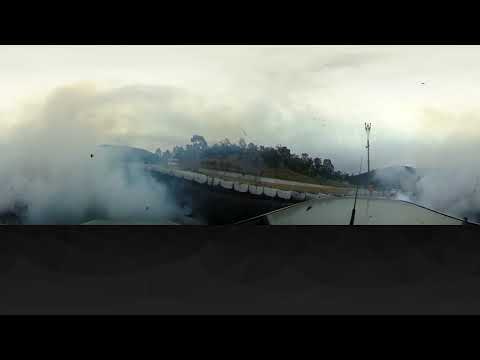The photograph appears to depict an outdoor scene featuring a dusty or smoky environment. Central to the image, there's a waterway, possibly a river, with what looks like a boat partially in the foreground on the right side. The water appears disturbed, with splashes possibly indicating movement or activity. To the left and right, large clouds of smoke or dust heavily obscure the view, rising and spreading across the scene. In the background, a landmass stretches across with a road running left to right, ending in a hilly terrain. Trees and grass are visible above the road, confirming the outdoor setting. The sky is overcast, showing a yellow or orange hue, potentially due to the smoke or dust in the air. The overall brightness suggests it could be early in the day.